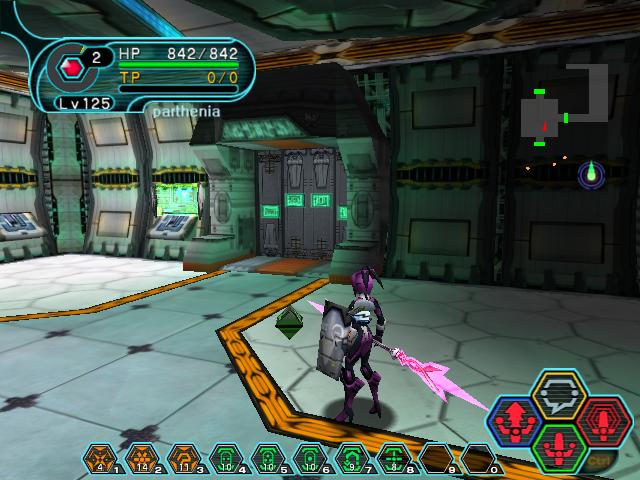In this screenshot from a video game, the interface elements are prominently displayed in the upper left corner. The player's stats indicate an HP of 842/842 and TP of 0/0. Below this, the level is shown as LV 125, and the player's character is named Parthenia. The setting appears to be inside a futuristic spaceship or metallic structure, characterized by metal walls and a distinctly advanced atmosphere. Centrally, there is a set of metal doors, adding to the sci-fi aesthetic. To the left, numerous computer screens with control panels and a sectioned-off white floor indicate a high-tech command area. 

In the foreground, towards the middle bottom right, the player's character is vividly detailed. She is adorned in a purple hat and high-heeled purple boots, wielding a large spear with a pink tip and pink accents, and carrying a gray rectangular shield. The bottom of the screen displays her inventory, detailing various items, weapons, and their respective quantities. This carefully crafted scene encapsulates the mix of exploration and combat integral to the game's experience.